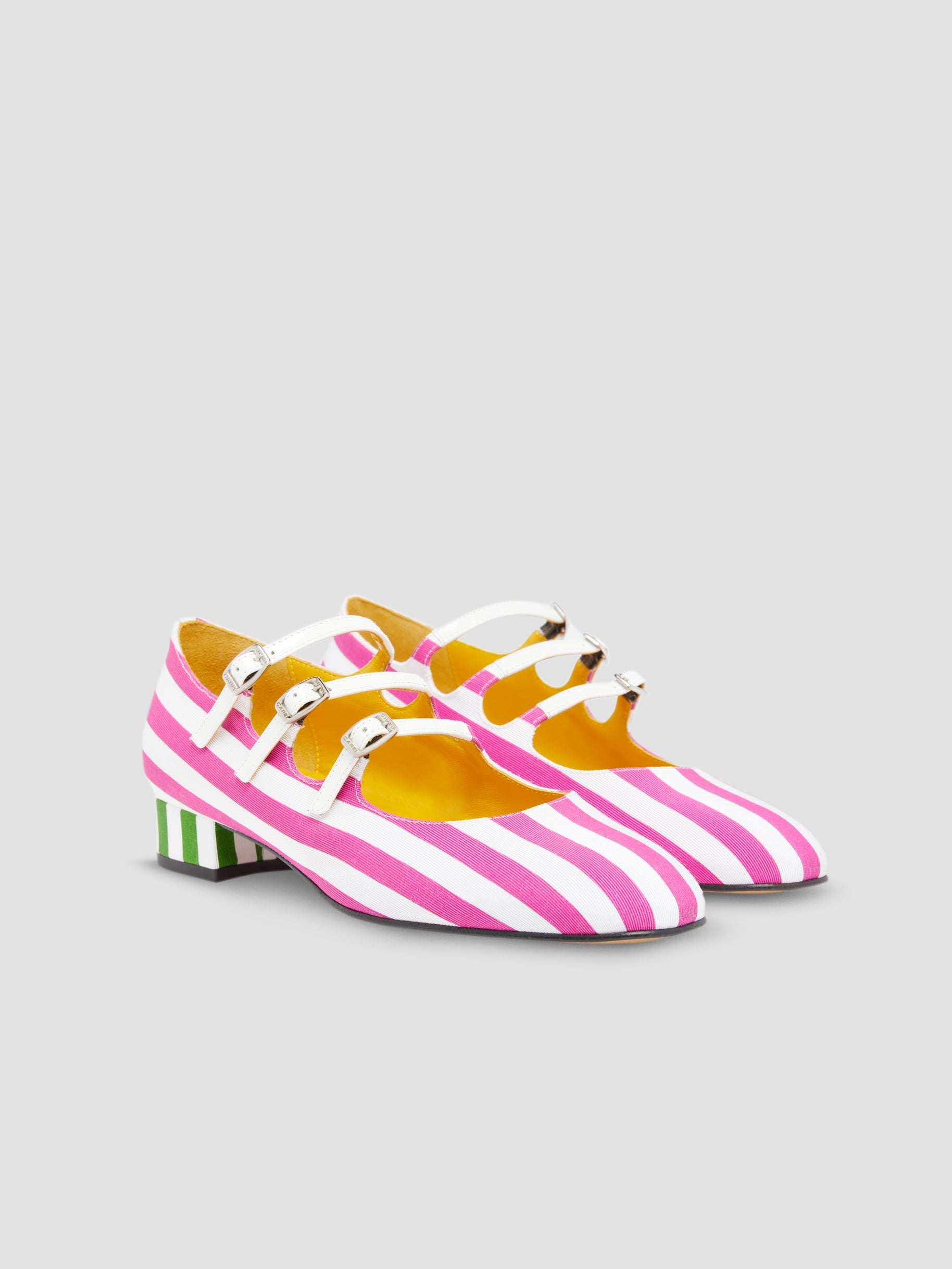This detailed image shows a pair of artistic women's Mary Jane shoes captured in a three-quarter view against a white background with flat lighting. The shoes are primarily white with bold hot pink vertical stripes running from heel to toe. They feature an intricate design with three silver buckles across the top of the foot and white straps. The heels of the shoes are mid-height, square-shaped, and adorned with striking green and black vertical stripes. The interior is a vibrant yellow, creating a stark contrast with the exterior. The material appears to be leather or pleather, adding to the high-fashion yet whimsical aesthetic of these unique, closed-toe shoes. The photograph's lack of shadow highlights the vivid colors and distinctive design elements, making the shoes resemble a piece of wearable art rather than everyday footwear.